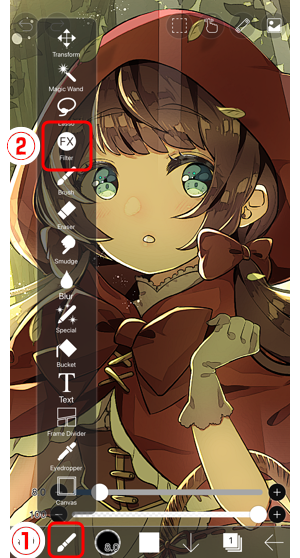The image is a screenshot from a graphic editing program featuring a vibrant, manga-style female character. She has large, striking green eyes, her lips shaped in a small 'O', and long brown hair styled into two lengthy braids, adorned with bows. The character is dressed in a 'Red Riding Hood' inspired outfit, comprising a deep red hood and cloak, a large bow on her chest, and a dress with closures down the front, complemented by gloves on her hands and a basket handle resting around her arm.

In the foreground, the software interface includes transparent overlay bars displaying an array of graphic editing tools. The number one position highlights an icon of a paintbrush, encased in a red square on the bottom menu. Number two marks the FX filter button, also highlighted similarly. Additional tools visible along the sidebar and bottom menu include options such as transform, magic wand, lasso, filter, brush, eraser, smudge, blur, special effects, bucket, text, frame divider, eyedropper, canvas, and directional arrows.